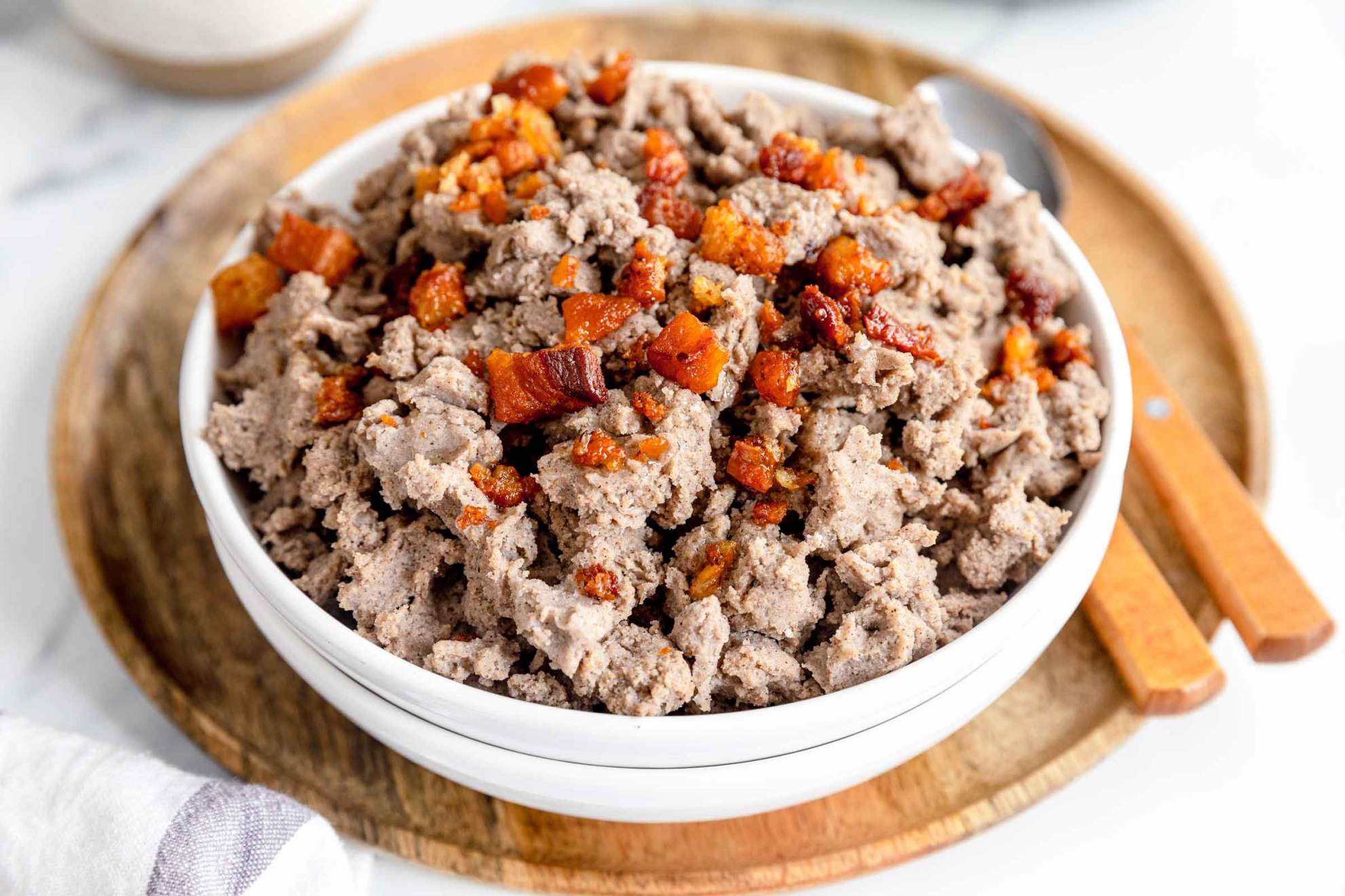This landscape-oriented, color photograph showcases a meticulously styled food scene reminiscent of high-quality food blogs or cookbooks. At the center of the image is a large, round wooden plate with a white bowl featuring a thin black border near its lip, placed on it. Inside the bowl is a mixture resembling crumbled ground meat in a grayish-brown tint, possibly hamburger, topped with chopped, cooked bacon and diced red grilled pepper. The bowl is accompanied by a spoon and a knife on the right side, both with metal surfaces and tan wooden handles. This arrangement rests on a gray and white marble-like surface adorned with a white and gray striped kitchen towel, capturing the essence of representational realism in food photography.